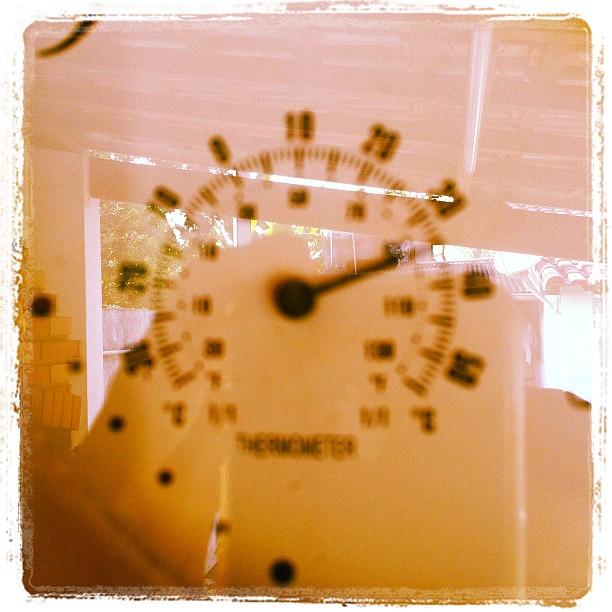The image depicts a uniquely designed gauge, reminiscent of a car's odometer, but with a distinctive and somewhat unconventional appearance. The display, dominated by yellow-amber tones and black text, intriguingly bears the word "thermometer." The gauge resembles a clock face, with large numerals encircling the outer edge and detailed calibrations marked around its perimeter. An indicator points to the upper right quadrant of the circular gauge, suggesting a specific reading.

The gauge appears to be set behind frosted glass, adding an element of translucency to the scene. This glass, intriguingly, has sections etched in pink with stripe patterns, enhancing its unique aesthetic. Beyond this glass, the view opens up to what seems to be a factory building. Through this semi-transparent barrier, one can discern lush bushes on the left side and roofing panels that glisten with water. Additionally, a calibrated roof and brickwork are visible, contributing to a layered backdrop that hints at an industrial setting.